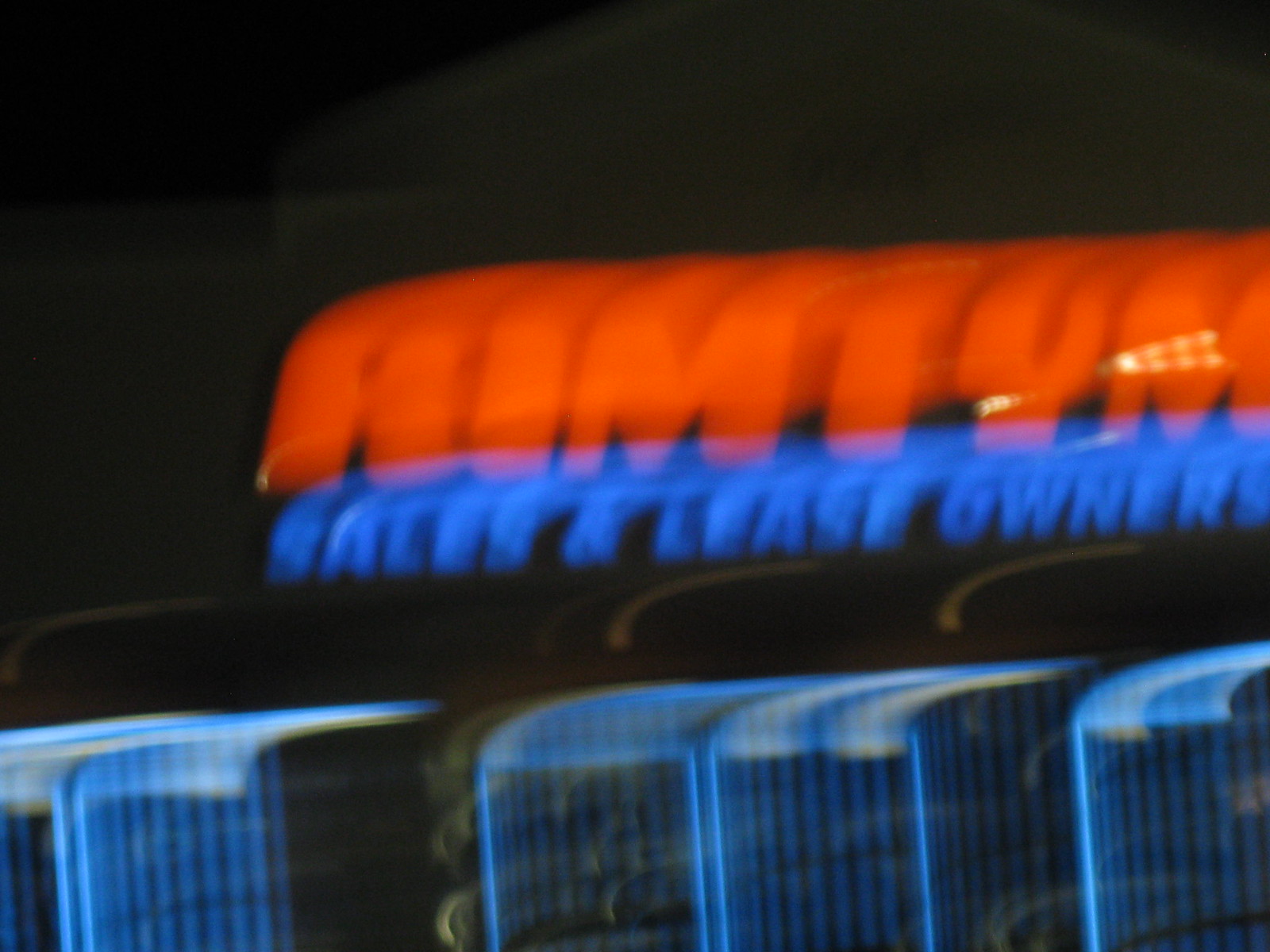The image depicts a nighttime scene featuring a sign that is partially obscured by darkness and motion blur. Dominating the center of the picture is a prominent red, illuminated sign with indistinct lettering, potentially reading "H-I-M-I-Y-M." Beneath this, blue text is faintly visible, spelling out "Sales and Lease Owners," and is also affected by motion blur. Below the blue text, thin, yellow lines can be seen, adding to the layered composition of the sign. Further down the sign, five blue-lit sections, resembling bars on a window, are noticeable, each displaying significant motion blur. The overall effect is a blend of colors and text, with the night and motion giving the sign an enigmatic and dynamic appearance.